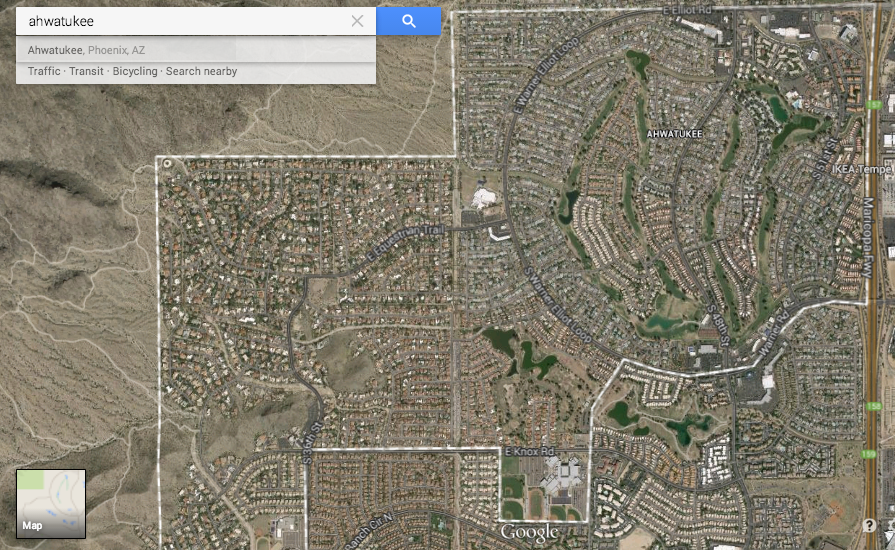A detailed satellite image of the Ahwatukee neighborhood in Phoenix, Arizona, displaying a complex network of maps, roads, and landmarks. In the top right corner, a blue square is labeled 'man-made glass.' The main image features a neighborhood densely populated with buildings, roads, and natural surroundings, including mountains. Various map markers indicate specific locations: 'A.L. Watukee,' 'Ikea,' and 'East Knox Road.' Among the distinguished routes are Warner Elliott Loop and a visible highway. 

At the very bottom right, a question mark is followed by 'Google,' hinting at the image source. Over on the bottom left, a white-outlined square showcases parts of the map, highlighting lakes and green fields at the center. Additionally, a freeway labeled 'Morris Groupa Freeway' is depicted towards the right side. The image offers a comprehensive overview of the neighborhood, combining elements of traffic, transit, and natural scenery to present a vivid depiction of the area.